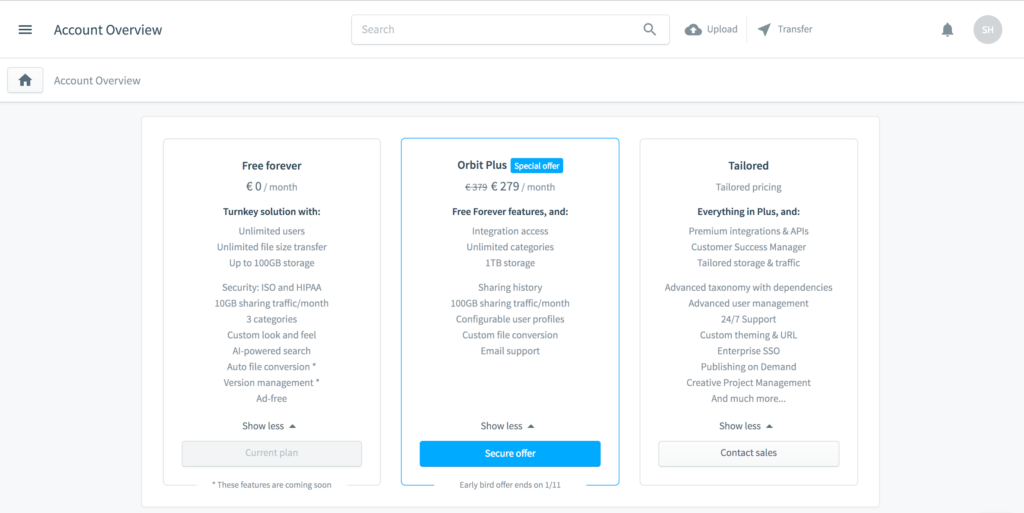In this image, we see the "Account Overview" page of a web application with a white background. At the top left, the page title "Account Overview" is displayed, accompanied by a menu icon. On the top right, there are several icons: a search bar, an upload feature, a transfer option, a notifications bell, and a user profile image.

The main section of the page is dedicated to three different subscription plans presented horizontally. 

1. **Free Forever:**
   - Cost: €0
   - Features:
     - Unlimited users
     - Unlimited file size
     - Transfer up to 100 GB
     - ISO and HIPAA security compliance
     - 10 GB sharing traffic
     - Customizable look and feel
     - AI-powered search
     - File conversion and version management
     - Upcoming features (marked as coming soon)
   - Button: "Current Plan" (currently selected)

2. **Orbit Plus:**
   - Special Offer: €279 (reduced from €379), highlighted with a blue background and white text
   - Features:
     - Includes all "Free Forever" features
     - Integration access
     - Unlimited categories
     - 1 TB of storage
     - Sharing history
     - 100 GB sharing traffic per month
     - Configurable user profiles
     - Custom file conversion
     - Email support with dedicated ninjas
   - Button: "Secure Offer" (highlighted with a blue outline)

3. **Tailored Plan:**
   - Premium plan with customized pricing
   - Features:
     - Premium integrations and APIs
     - Customer success manager
     - Tailored storage and traffic options
     - Advanced taxonomy and dependencies
     - Advanced user management
     - 24/7 support
     - Custom timing and URL options
     - Enterprise Single Sign-On (SSO)
     - Publishing on-demand
     - Creative project management
     - Additional premium features
   - Button: "Contact Sales" (currently greyed out)

Each plan offers a progressively more comprehensive set of features tailored to different user needs, from individual to enterprise-level requirements.